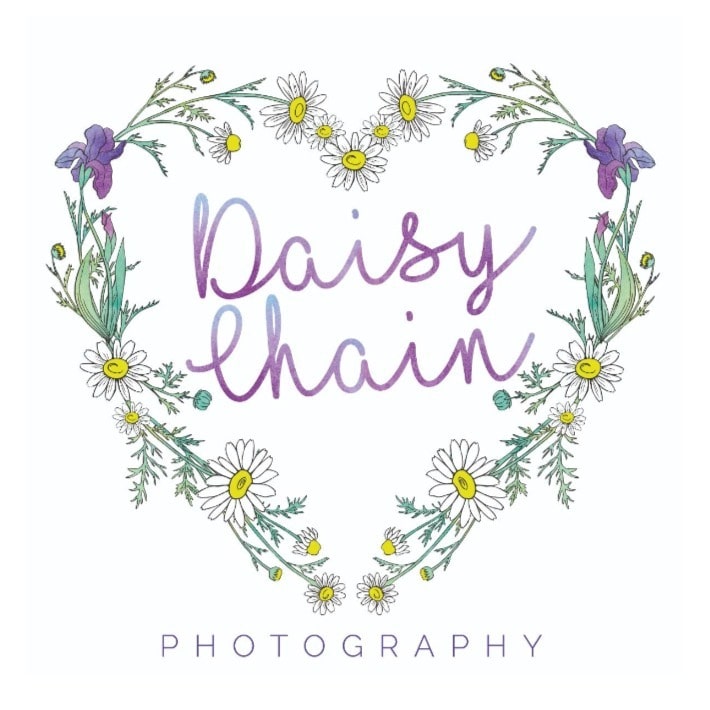The image depicts a logo for a photography studio named "Daisy Chain Photography." The central design features a heart shape formed by a combination of animated flowers, predominantly white daisies with yellow centers and smaller purple flowers, possibly irises. Inside this floral heart, the words "Daisy Chain" are elegantly written in a purple gradient cursive font, with "Daisy" on the first line and "Chain" below it. Both the 'D' in Daisy and the 'C' in Chain are capitalized. Underneath the floral heart and the cursive writing, the word "PHOTOGRAPHY" is displayed in capitalized, thin block letters in a dark hue, potentially blue or purple. The entire logo is set against a plain white background, emphasizing the colorful floral heart and the elegant lettering.